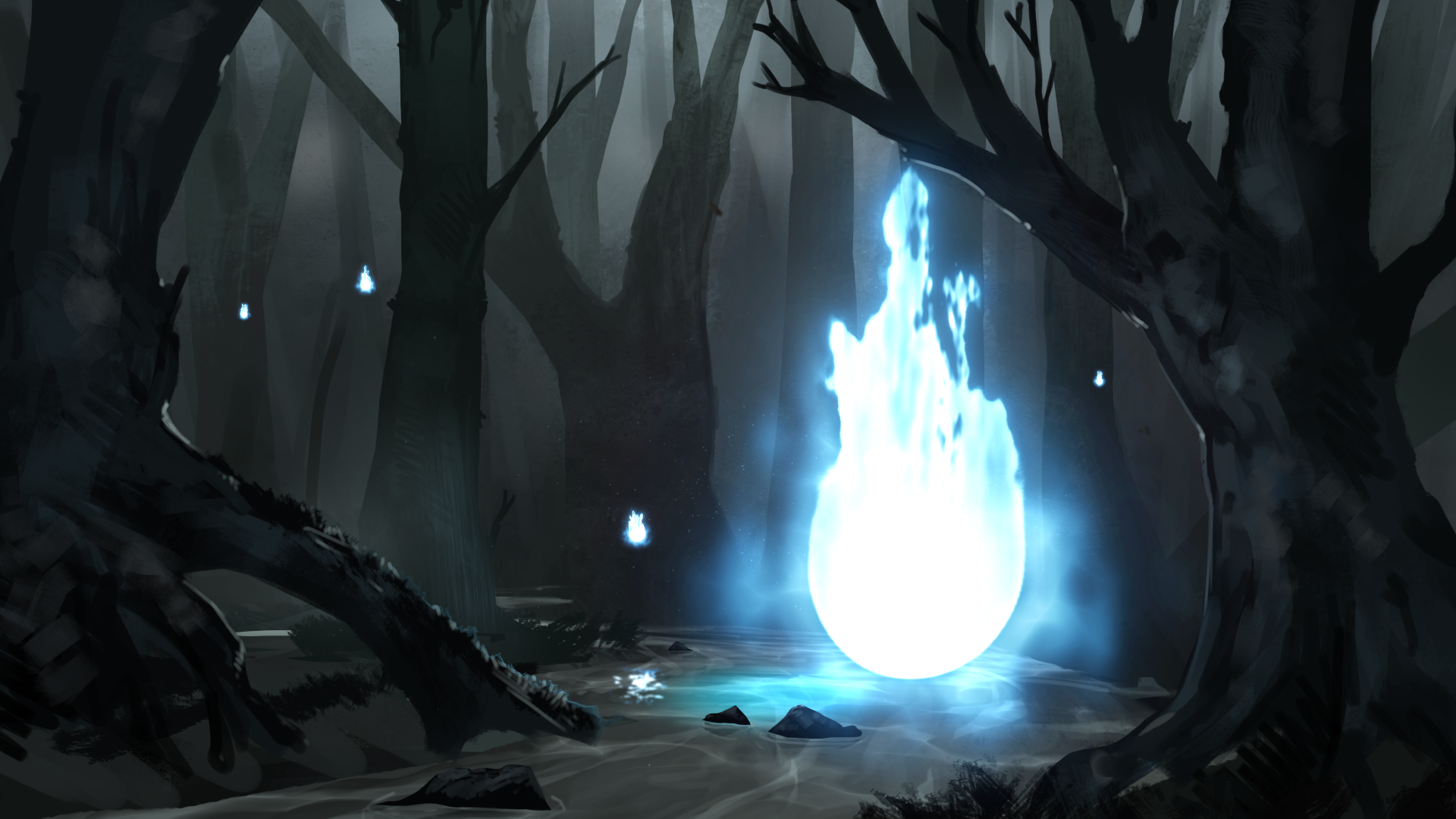In this eerie, dark, and gloomy drawing of a forest, the background is shrouded in gray fog, enhancing the overall spooky atmosphere. Black tree trunks and large branches dominate the scene, devoid of leaves and creating a skeletal appearance. The focal point is a large, bright white orb with blue streaks and flames radiating from the top, located just right of the center. This orb glows intensely, casting a blue aura that illuminates the immediate area around it. Surrounding this central orb are several smaller orbs floating in the background, positioned amongst the trees—one to the left of the large orb, two towards the middle left, and another as you move towards the right. Additionally, two rocks are situated in front of the main orb, contributing to the scene's unsettling ambiance. The combined effect of the fog, stark trees, and glowing orbs creates a haunting, almost spectral forest scene reminiscent of a Halloween setting.